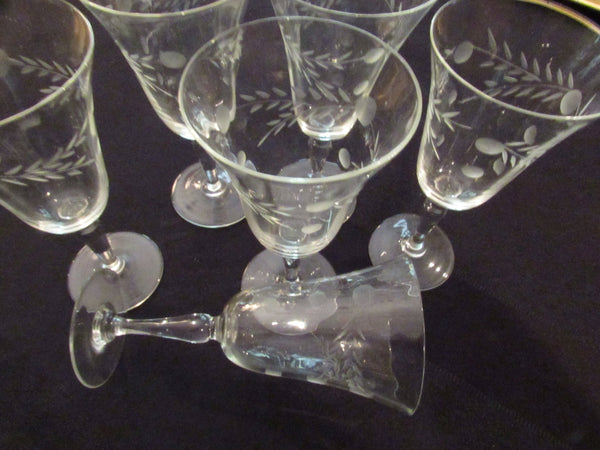The image portrays a set of six antique-style wine glasses arranged on a dark, possibly black tablecloth or surface. Five of the glasses stand upright, arrayed with four forming a row behind one that is slightly forward. The sixth glass is laid down in the foreground. These glasses feature an elegant design that includes etched patterns resembling leaves and small berries or fruit, most likely suggestive of grapevines. Their clear, slightly musty appearance hints at age or a need for cleaning. The angle of the shot is from above, making the openings of the glasses look larger. The overall scene encapsulates a vintage charm against a stark background.